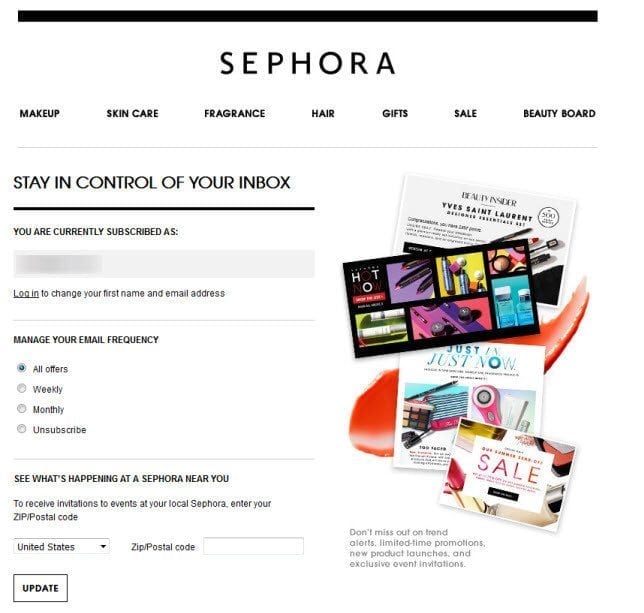The image features a clean, organized layout with a predominantly white background. At the top, there is a black bar, and prominently centered below it is the word "SEPHORA" in bold, capital letters. Beneath the title, a horizontal menu displays various categories: "Make-Up," "Skin Care," "Fragrance," "Hair," "Gifts," "Sale," and "Beauty Board." 

Following the menu, a grey line separates the header from the body of the content. The main section begins with the text "Stay in control of your inbox," highlighted by an underline. Beneath this, it states, "You are currently subscribed as," followed by a blurred-out grey box containing subscription details. Another line of text prompts users to "Log in"—underlined—to change their first name and email address.

A minor grey line introduces the next set of options: "Manage your email frequency." Here, four opt-in options are listed vertically with clickable boxes: "All Offers" (selected), "Weekly," "Monthly," and "Unsubscribe." 

Toward the bottom, another grey line precedes the text "See what's happening at a Sephora near you." This section invites users to enter their zip/postal code in an empty box, adjacent to a drop-down menu set to "United States" by default. To the right, there's text encouraging users not to miss trend alerts, limited-time promotions, new product launches, and exclusive event invitations.

On the left, below all this information, there's an "Update" button. 

The right-hand side of the image is filled with vibrant pictures of makeup, various flyers, and a "Sale" tag, providing a visually appealing balance to the left-aligned text-heavy content.